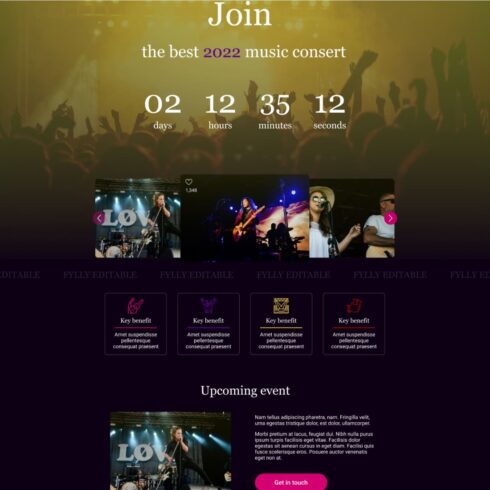Join us for the Best 2022 Music Concert! The countdown is on with just 02 days, 12 hours, 35 minutes, and 12 seconds remaining. The vibrant background captures the electrifying atmosphere of the event, featuring a bustling stage area lit by bright lights. The crowd is energy-filled, with hands raised high in excitement. 

The images showcase dynamic concert moments: 
- A performer gripping a microphone with dramatic stage lights behind them.
- A central figure playing the guitar, dressed in a striking red jacket.
- A woman artist, coolly working the stage in sunglasses and a hat, standing confidently in front of her microphone.

Below these snapshots is the announcement for the upcoming event, highlighted in white text, alongside another musical artist on stage, bathed in blue lights, dressed in black and holding a microphone. Adjacent to this is a detailed paragraph of text in white, providing further information about the event. 

Finally, a prompt in pink at the bottom encourages you to "Get in Touch" for more details. Don't miss out on this unforgettable musical experience!